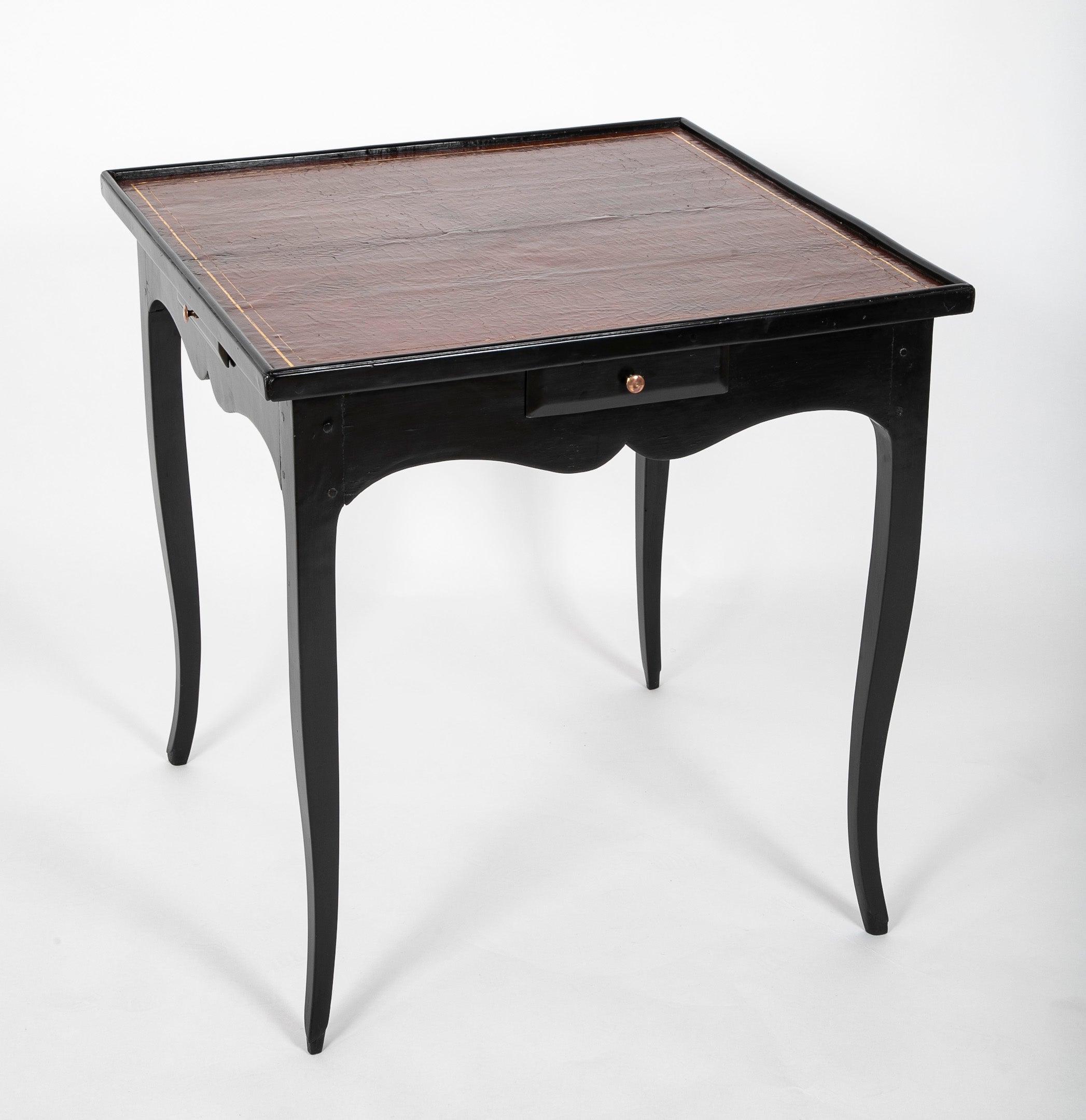This is an enlarged, up-close image of an elegant side table, set against a completely white background, with no text or other elements present. The table features four thin, subtly wavy legs that are quite long. The table structure, lacquered in black paint, also showcases a distinctive, intricate design beneath the tabletop: a harmonious combination of curves and mounds that add a touch of sophistication. The tabletop itself is a dark brown color, slightly wider than the table’s body, possibly due to the type of wood or a tightly adhered fabric used. In the center of the table, there is a faux drawer adorned with a small, gold-colored knob, which, despite its appearance, does not function as a real drawer. The overall design exudes a certain level of fanciness, highlighted by the play of shadows pointing towards the top left, indicating the light source is from the right of the image.